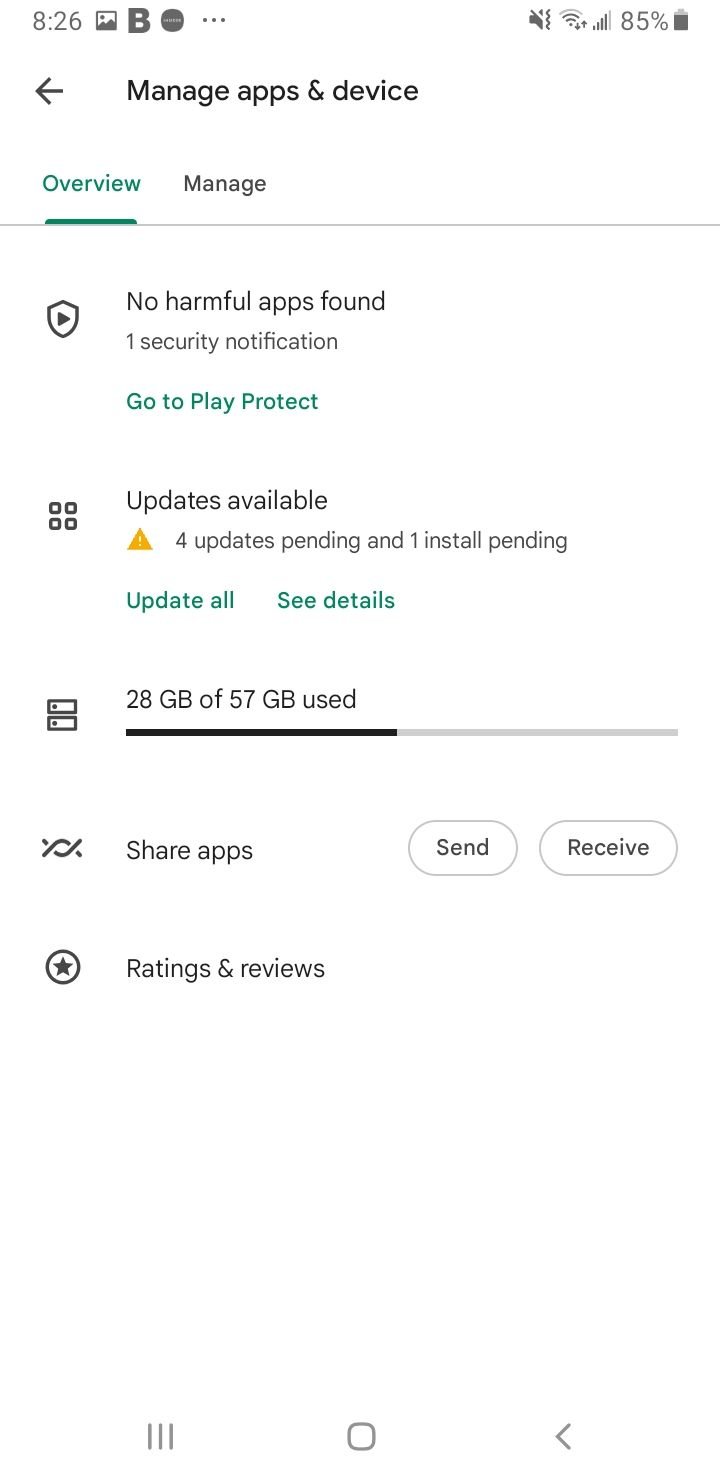The image shows a white background with a detailed screen capture from a device, presumably a smartphone. In the top left-hand corner, there is a gray rectangle. On the right side of the gray rectangle, there is a small amount of space followed by the time displayed as "8:26". 

Adjacent to the time, there is a gray "B", a gray circle containing an illegible white word, and three gray dots. Further along, the battery icon indicates the phone is charged at 85%. 

Below this top section, a black arrow points to the left, next to the text "Manage Apps and Devices" written in black. After some space, on the next line, the word "Overview" appears, followed by a teal underline that stretches underneath it. To the right of this section, the word "Manage" can be seen. 

A line spans across the width of the screen, below which it reads "No harmful apps found" and "One security notification" in gray. This is followed by a teal-colored prompt that reads "Go to Play Protect".

Further down, the text "Updates available" is shown, accompanied by a yellow triangle containing a white exclamation point. The gray text below states "Four updates pending and one install pending".

Following this, in teal, the option "Update all" is displayed, with "Details" also present nearby. At the very bottom, the storage information indicates "28 GB of 57 GB used", underneath which there is a mention of "Share apps and ratings and reviews".

This detailed description captures the exact layout and contents of the screen for informative and visual reference.